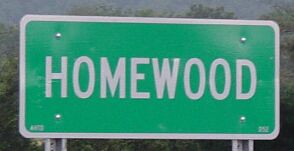In the background of this image, the sky is slightly visible and appears gray. Green tree and bush tops can be seen. Dominating the scene are two hollow, metal posts with a V-shaped back, both supporting a rectangular sign. The sign, trimmed in silver, prominently displays the word "Homewood" in silver lettering against a green backdrop, secured by four visible screws.